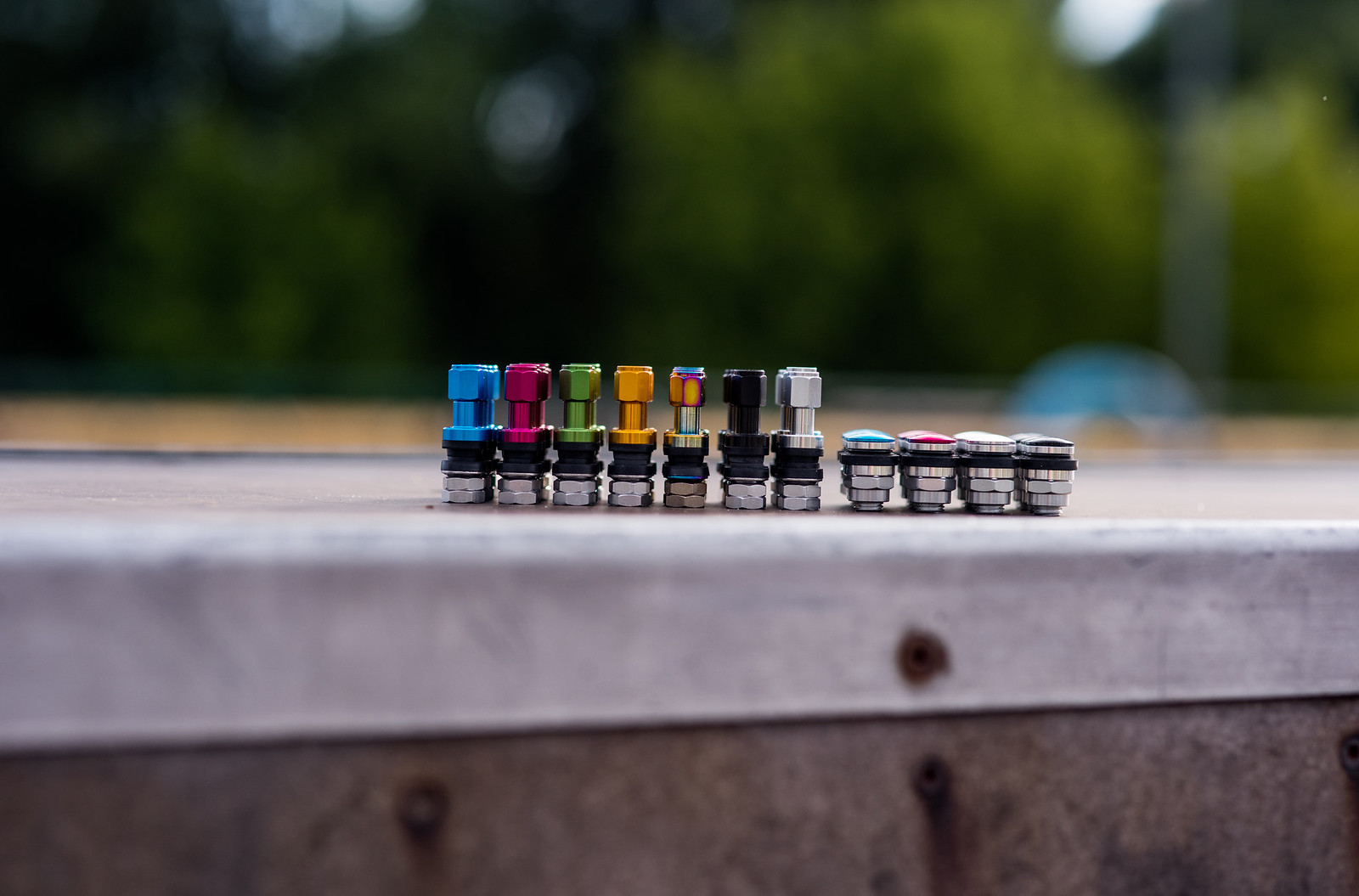The image is a color photo capturing the top of what appears to be a metal roof or a ledge, with a detailed focus on a series of metal fittings or attachments that resemble bolts. These fittings are lined up meticulously in a straight line, with a total of eleven visible pieces. The first seven fittings from left to right are taller and feature anodized colors: blue, pink, green, yellow, a multicolored piece with yellow and pink, black, and plain silver. The shorter four fittings to the right have tops that are blue, pink, white, and black. The base of each fitting is a silver color, resembling stainless steel or chrome, while some parts appear to be bronze. The background is blurred but showcases greenery and trees, suggesting the photo was taken outdoors in a park-like setting. This well-organized array of colored metal fittings forms the central focus, highlighting their vibrant, neon hues against the metallic base and the natural backdrop.